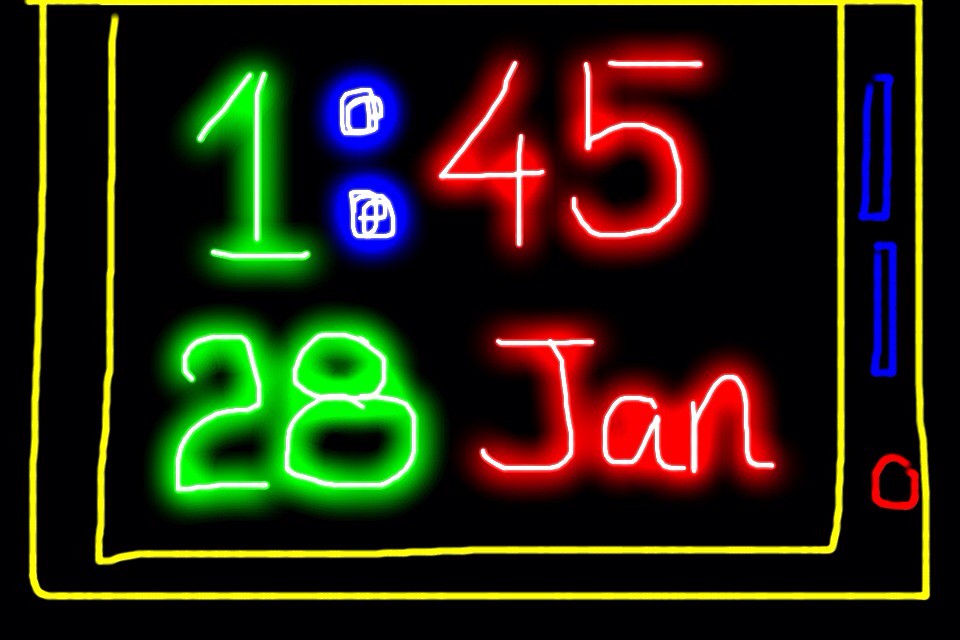The image features a digital neon sign against a black background. It is framed by two thin yellow square outlines which evoke the shape of an old-style television. Nested between these yellow lines on the right are two vertically aligned bright blue rectangles, with a red circle directly below them. Centrally located within the inner yellow square, the number "1" in neon green with white accents is displayed prominently, with "28" in green and white beneath it. To the right of the "1" are two blue circles with white squiggly lines inside them. Further right, "45" in a red neon hue with white accents is displayed, and below it, also in red with white, is the abbreviation "JAN." The combination of colors and shapes suggests a blend of time and date information, possibly representative of a clock displaying "1:45" and the date "28 JAN."